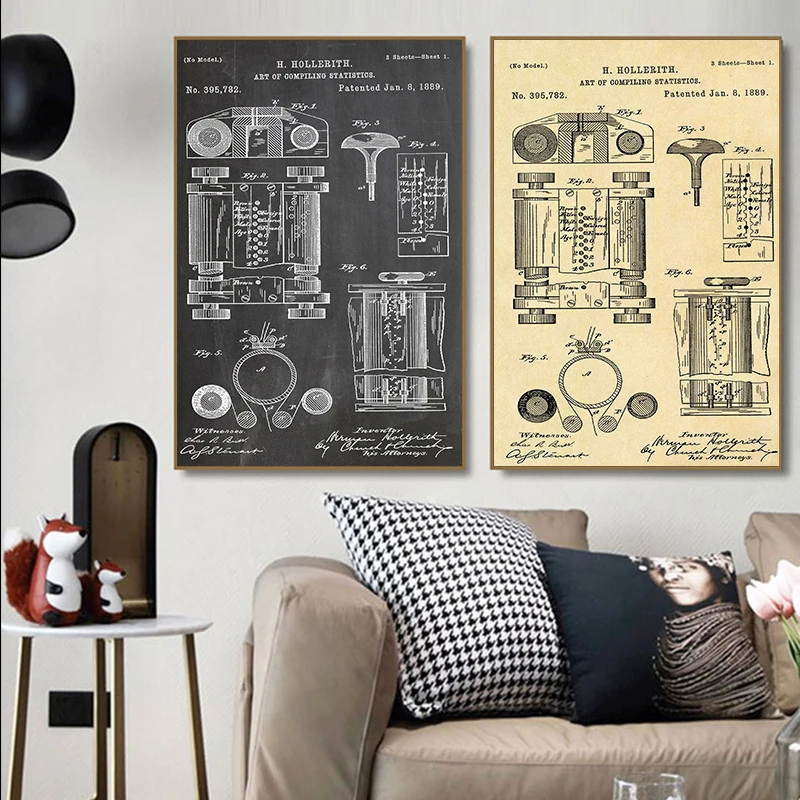The photograph depicts a cozy living room with a focal point on two large posters mounted on a white wall. Both posters illustrate the same detailed diagram, likely a patent, dated January 8th, 1889, attributed to H. Hollerith. The left poster features a dark gray background with white schematic illustrations of the device, while the right poster displays the same design against a yellow background with black linework. Beneath these intriguing art pieces, a tan couch adorned with a houndstooth black and white pillow and a black pillow featuring a female face invites comfort. To the left of the couch, an end table holds two charming figurine foxes and a vase with tulips, contributing to the room's aesthetic. A tall lamp with dual globes peeks in from the top left, casting a warm glow over the thoughtfully curated space.